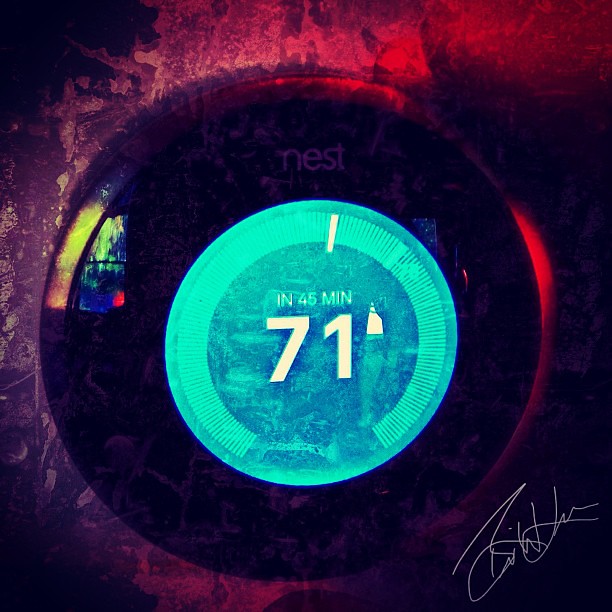The image features a digital Nest thermostat prominently displayed in the center. The face of the thermostat is illuminated in a glowing neon blue, creating a striking visual effect. The thermostat reads "In 45 minutes" in light blue text at the top, with the temperature setting displayed in bold white numbers as "71". The Nest logo appears at the top of the device in white text. 

There are reflective elements on the thermostat's surface, suggesting someone took the photo, adding a subtle human presence to the composition. Surrounding the smoothly contoured black body of the thermostat are artistic digital flourishes: to the left, a petal-like shape with a gradient of yellow to green, and edges tinged with blue and red highlights.

The background contrasts vividly against the thermostat, divided into bold colors and textures. The right side of the background is predominantly red with splashes and streaks of white paint, creating a dynamic, almost chaotic feel. Conversely, the left side of the background is swathed in rich purple hues with scattered white splotches, offering a stark yet complementary juxtaposition to the red. A signature in white can be found at the bottom right corner, hinting at the artistic nature of the piece and leaving ambiguity as to whether the image is a photograph with heavy digital manipulation or a painting mimicking photographic realism.